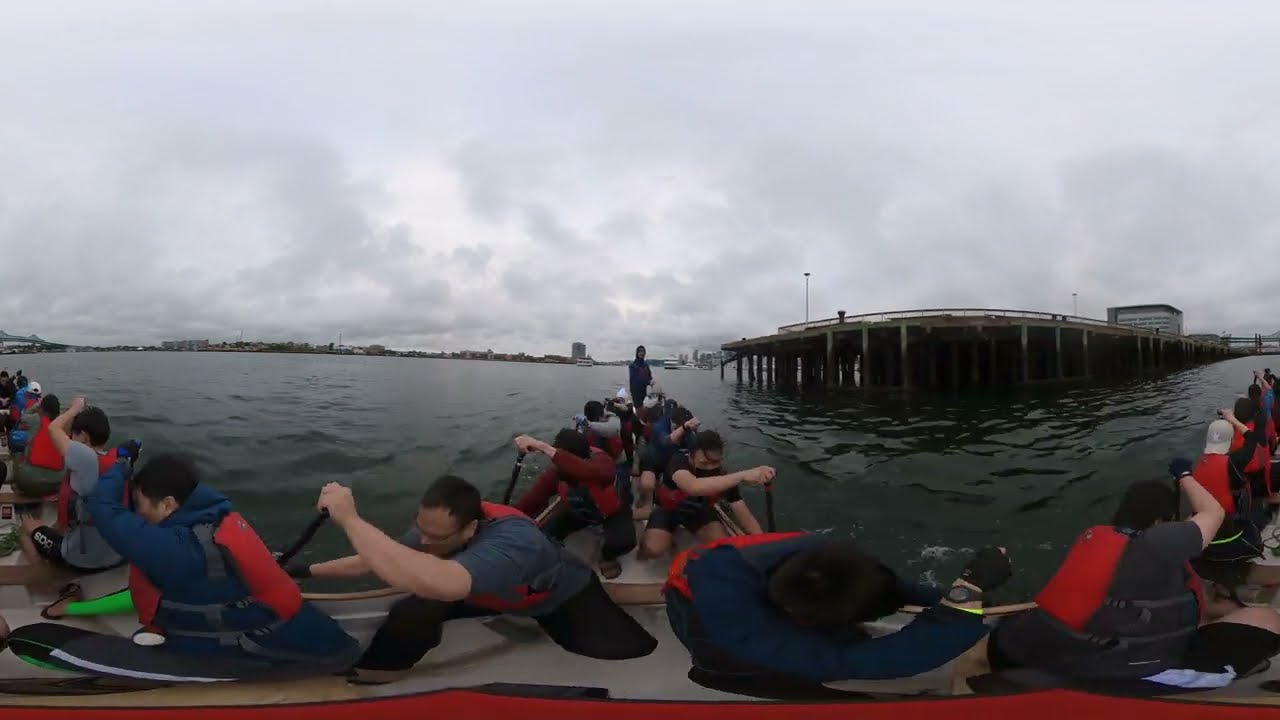The image depicts an outdoor scene set on a large, greenish body of water, possibly a lake or river, with ripples indicating movement. It’s taken from an angle that makes it appear almost spherical, like through a fisheye lens or VR goggles. The foreground is filled with several elongated, narrow canoes, each wide enough for a single person. Canoes are primarily tan, though one features a distinctive red bottom. 

Groups of people are actively rowing these canoes with noticeable effort. Among them, each person is equipped with a red life vest and paddles. They're dressed in a variety of clothing, including blue, gray, red, and sometimes neon green garments. A standout detail includes a person in the bottom left wearing neon green leggings. Most rowers are seated, but one individual in a blue hoodie and dark pants stands at the back of a canoe, providing a focal point amidst the activity. 

The background showcases a subdued sky with gray and white clouds and a modest city skyline with various buildings. A bridge or elevated road stretches across the water, characterized by its cement posts, adding architectural interest and context to the scene. The atmosphere is busy yet serene, reflecting a communal or competitive rowing event under the daytime cloud-cover.